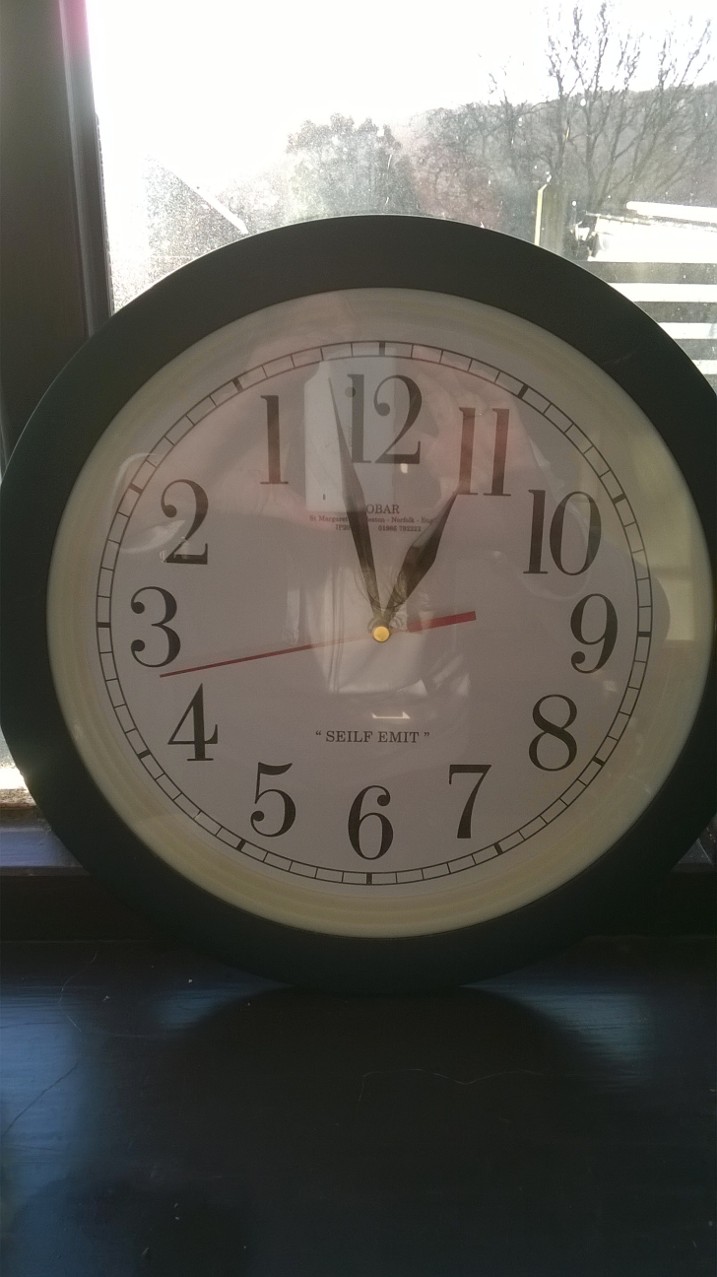This photograph captures a unique clock with a contemporary design. The clock features a sleek, glossy, black circular frame and a face with a pale yellow center surrounded by white. Notably, the clock runs counterclockwise, with the numbers arranged in reverse order—12, 11, 10, 9, and so forth. The time displayed is approximately 11:50, based on the large hand positioned between 1 and 12, and the small hand resting slightly on the 11. A red second hand stands out against the clock face, adding a touch of color.

The clock is placed on a dark, possibly black-stained wooden cabinet or dresser. Behind the clock, there is a window through which one can see a white fence and some trees, hinting at a serene yard beyond. The reflection in the clock's glass reveals the photographer, who appears to be wearing a short-sleeved white shirt. The intricate details and reflections add layers of interest to this seemingly simple yet captivating image.